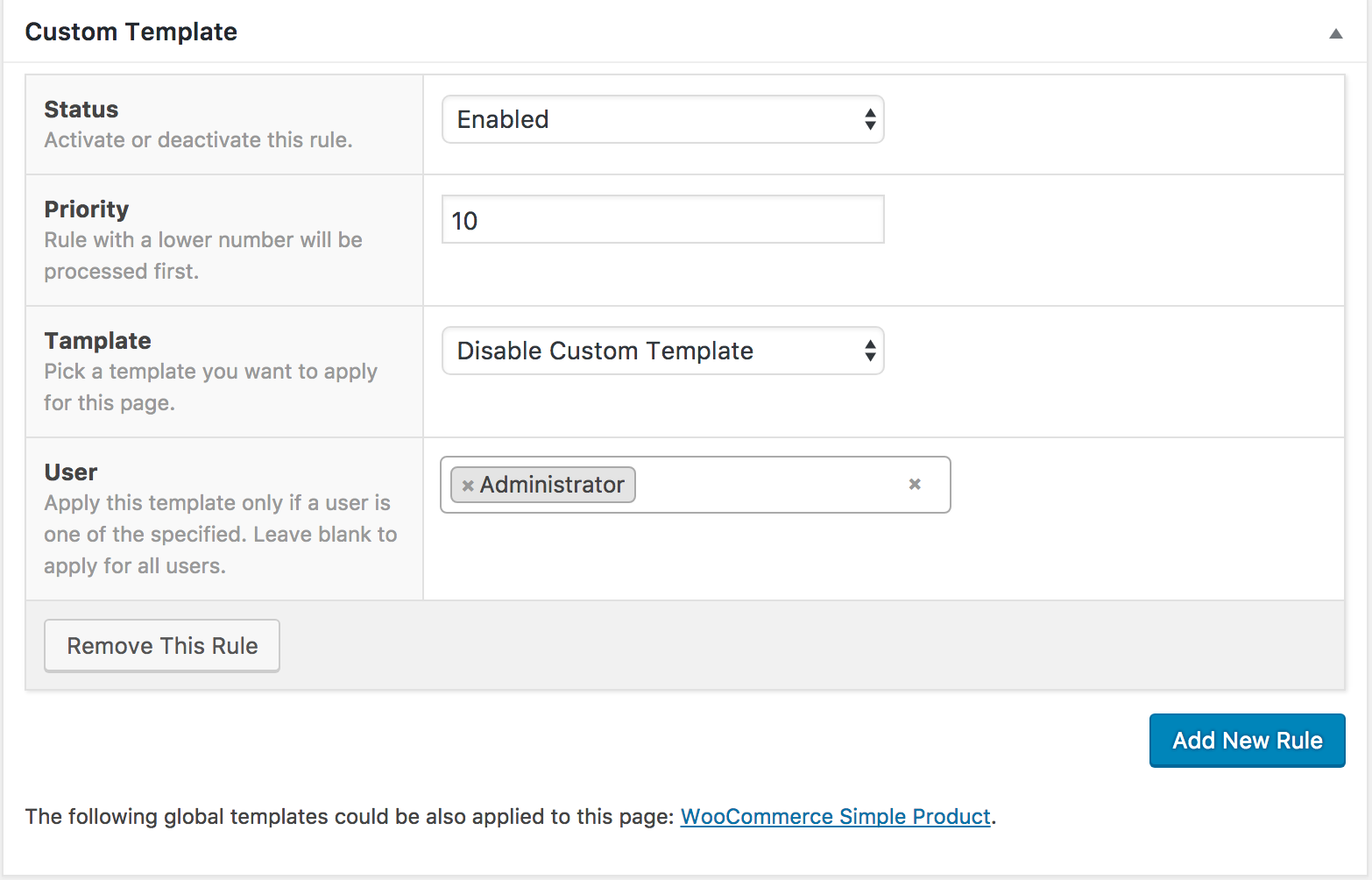The screenshot of the desktop application showcases the interface for custom template management. In the top left corner, the header reads "Custom Template." To its right, there's an icon resembling an upwards-facing arrow. Below the header, a section titled "Status" offers the option to activate or deactivate the rule, accompanied by a drop-down menu labeled "Enabled."

Directly under the "Status" section is "Priority," with a note clarifying that rules with lower numbers will be processed first. The priority level for this rule is set to "10." Further down, the "Template" section allows users to select a template to apply to the page, with an option to "Disable Custom Template" located to the right, accessible via another drop-down menu.

The "User" section enables the assignment of templates to specific users. The text field to the right of this section contains the word "Administrator" within a grey-shaded rectangle, along with a clickable "X" for removal. Users can drag and drop or manually add user types into this field.

Below the "User" section is a white rectangular button labeled "Remove this Rule," set against a light grey background. Towards the bottom right is a prominent blue button that reads "Add New Rule." 

In the bottom left corner, a description mentions that global templates can also be applied to the page, highlighting "WooCommerce Simple Product" as a clickable blue hyperlink.